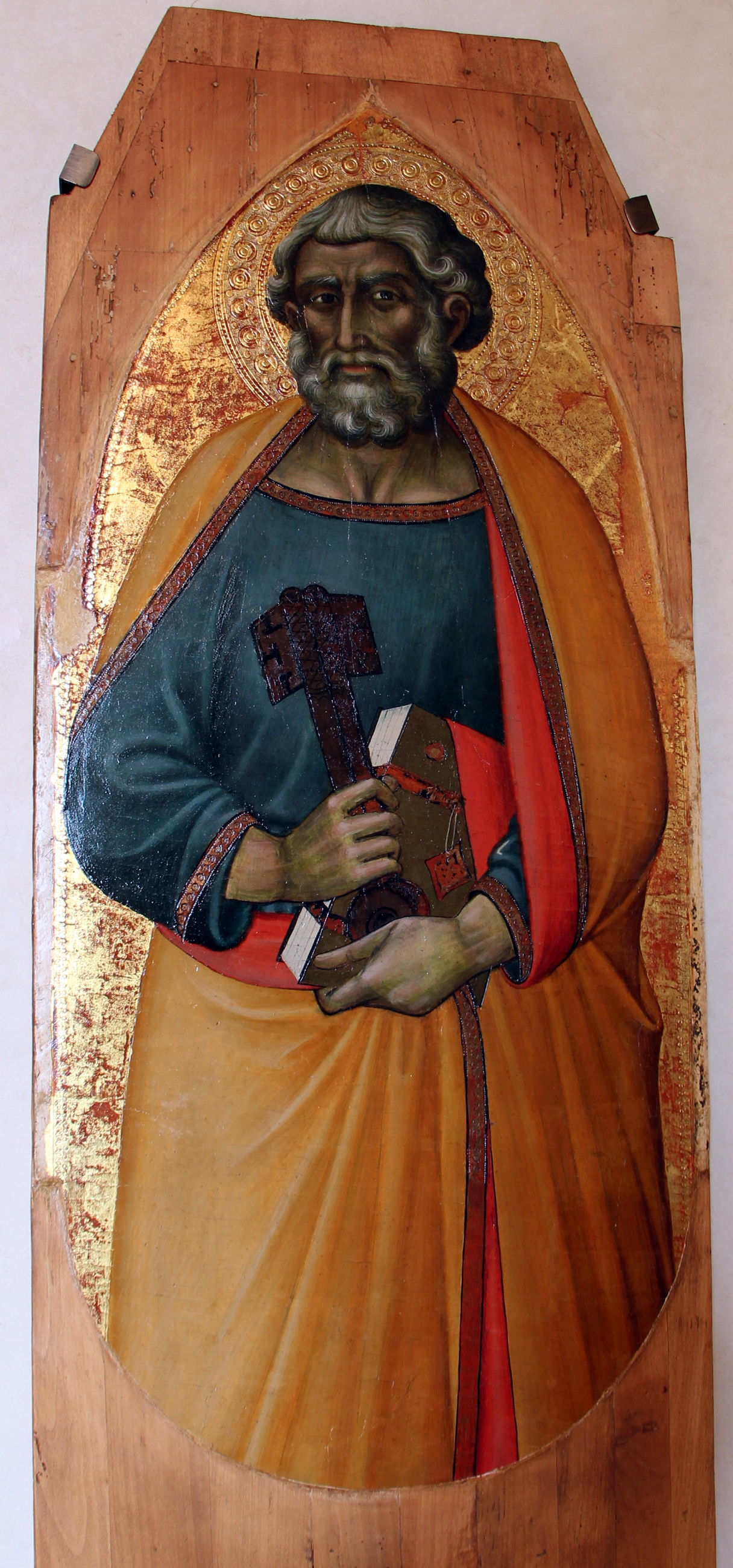This detailed painting depicts a religious icon, prominently presented on a large wooden panel with a background made of pressed gold leaf and accented with metallic golds and oranges. The focal point is an elderly man with a white and gray beard and abundant hair. He is clothed in a striking gold robe with a red lining, and beneath it, he wears a greenish-blue shirt with reddish borders. The intricate robe features a long sleeve that resembles a sling, in which his left hand rests. His right hand grips a black hammer or scepter. His left hand also holds a heavy book with a brown cover adorned with a prominent red stripe. The image is marked by vivid detail and bright colors, indicating its religious significance, likely originating from a church setting. The background extends to the light-colored wooden panel on which this refined artwork is created.